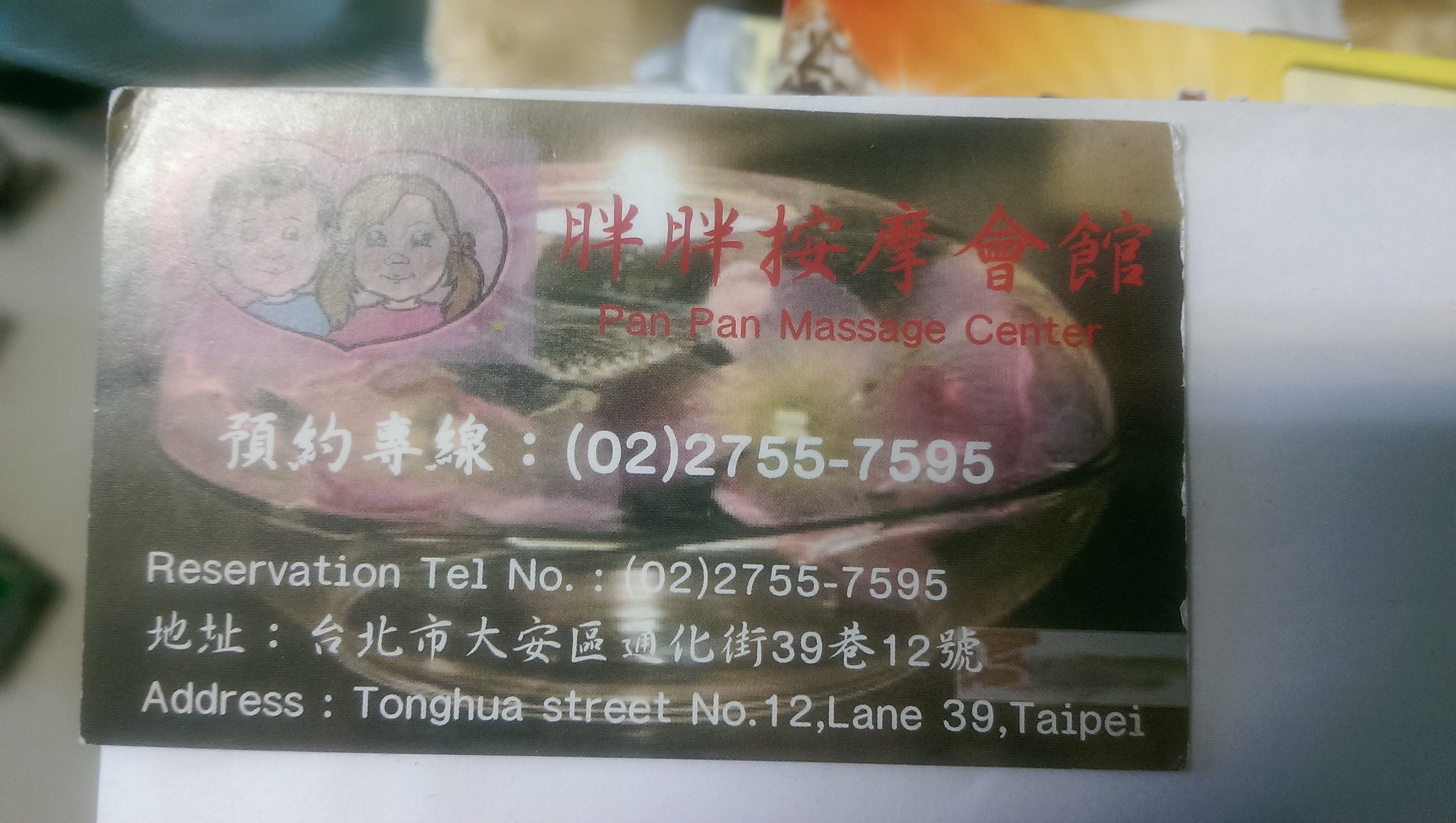The photograph depicts a business card for a massage center, resting on a blurred piece of white paper. The background shows a faint image of a glass bowl containing items that resemble massage stones, adding a spa-like ambiance. Positioned at the top left of the card, there's a heart-shaped logo featuring cartoon characters of a boy in a blue shirt and a girl in a pink shirt. In the upper right corner, there are Chinese characters in red, followed by the English name "Pan Pan Massage Center." Beneath this, additional details are provided in both Chinese and English, including the phone number 02-2755-7595. The card also lists three rows of information in white text: reservation details, towel number, and another mention of the telephone number, alongside more Chinese characters and an address. The address is specified as Tanghua Street, number 12, lane 39, Taipei.